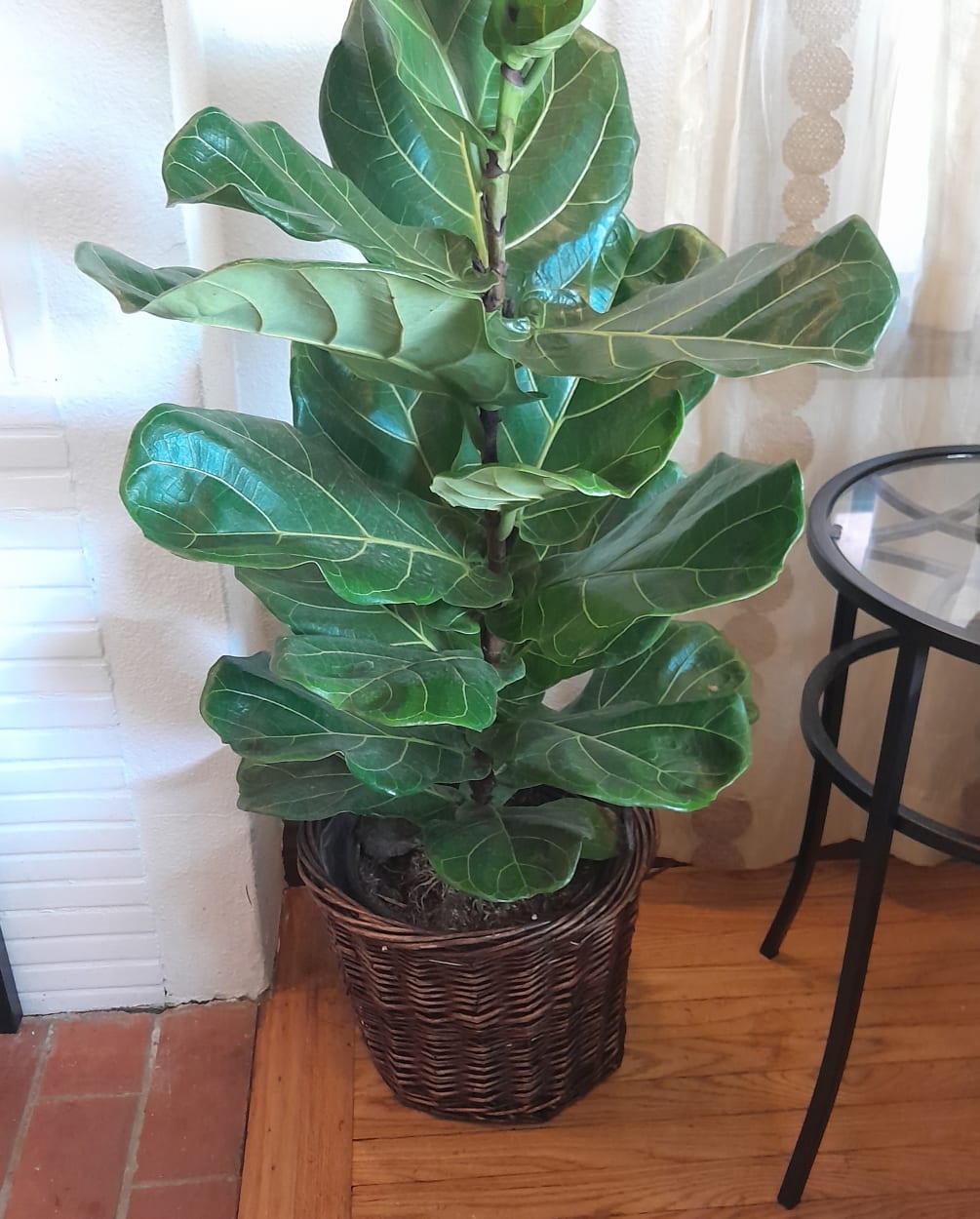This detailed color photograph captures a thriving fiddle leaf fig plant. The robust plant is teeming with dark, glossy, and substantial leaves, each marked by prominent light green veins that extend from central stems, giving the plant a lush and vibrant appearance. It is housed in an elegant dark woven rattan basket, which includes a plastic pot for added stability. The fiddle leaf fig stands impressively tall, reaching about halfway up the white wall behind it. It is situated on a floor that transitions from honey oak on the right to brick on the left, reflecting a stylish yet cozy interior setting. To the right of the plant, there is a small side table with an iron frame and a glass top, positioned under a window draped with sheer curtains. The combination of these elements, including the intricate details of the plant’s large, oval, and curvy leaves, creates a scene of serene natural beauty within a modern home setting.